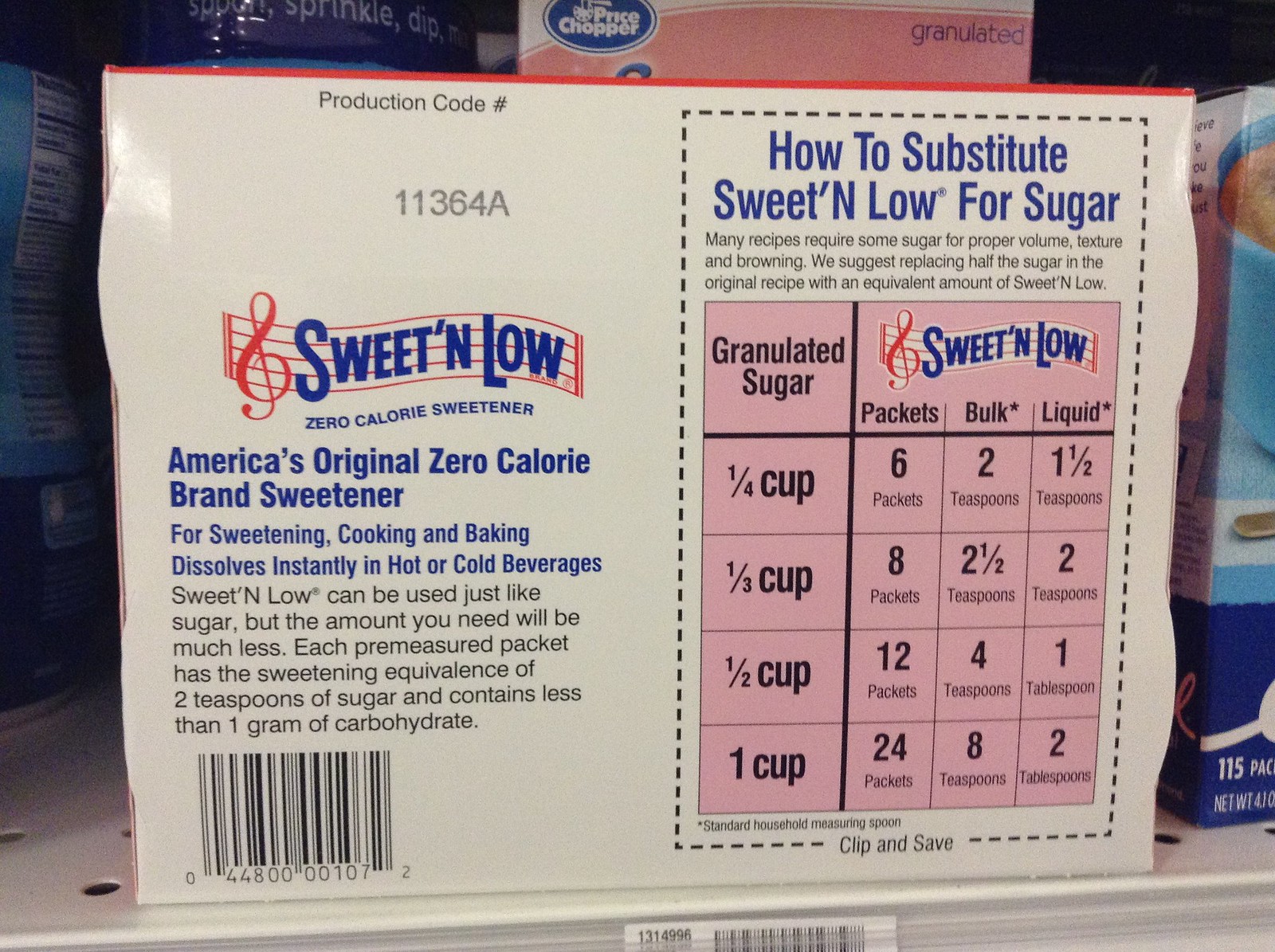This is a detailed close-up photograph taken in a retail store, showcasing a package of Sweet'n Low, America's original zero-calorie branded sweetener. The white rectangular package appears slightly grey due to low lighting and is positioned on a shelf with black perforations and a visible barcode label at the bottom edge. The left side of the package features the Sweet'n Low musical logo, with descriptive text stating it’s ideal for sweetening, cooking, and baking, and that it dissolves instantly in hot or cold beverages. Additional text elaborates on the product's features, including a production code number 11364A and the nutritional detail that each pre-measured packet has the sweetening equivalent of 2 teaspoons of sugar and contains less than 1 gram of carbohydrates. The right side highlights a serrated cutout section labeled "Clip and Save," featuring a table on a pink background that provides specific substitution instructions for replacing sugar with Sweet'n Low in various measurements. Just behind this package, another similarly branded package in pink and blue is partially visible, and to the right, the edge of another blue and white food carton can be seen.